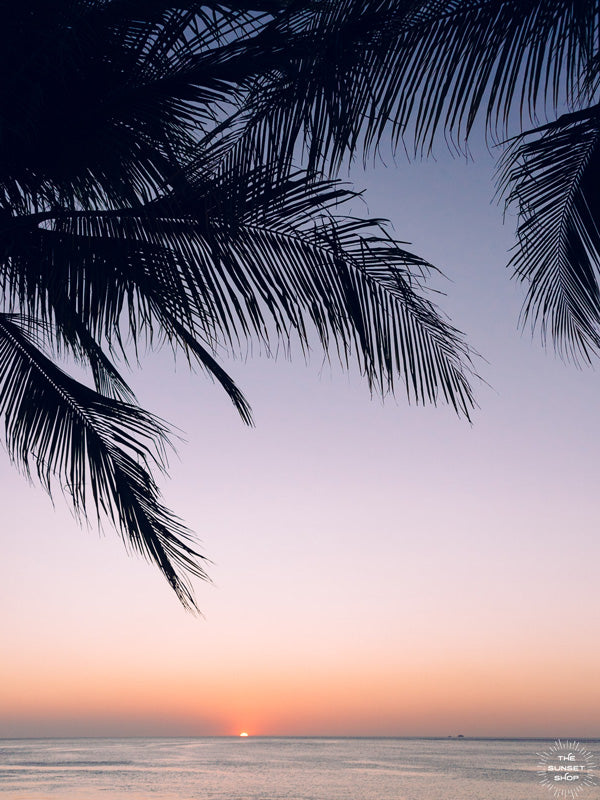The image captures a stunning tropical sunset over a vast ocean, viewed presumably from a beach. The horizon showcases the sun, half-set, illuminating the scene with a gradient sky - dark orange and reddish hues at the bottom, transitioning to lighter yellows, and finally a deepening blue as it ascends. Silhouetted against this breathtaking backdrop are dark palm trees; notably, one set with four visible fronds on the left and another tree on the top right corner, both contributing to the serene scene. In the distant water, there's a small indistinct shape that could be an islet or a boat, with gentle, clear waves visible on the ocean's surface. A white logo of a sun with the text "The Sunset Shop" adorns the bottom right, with artistic touches on the letters. The overall composition beautifully blends the natural splendor of the ocean and sunset sky, framed by the elegant silhouettes of palm fronds.